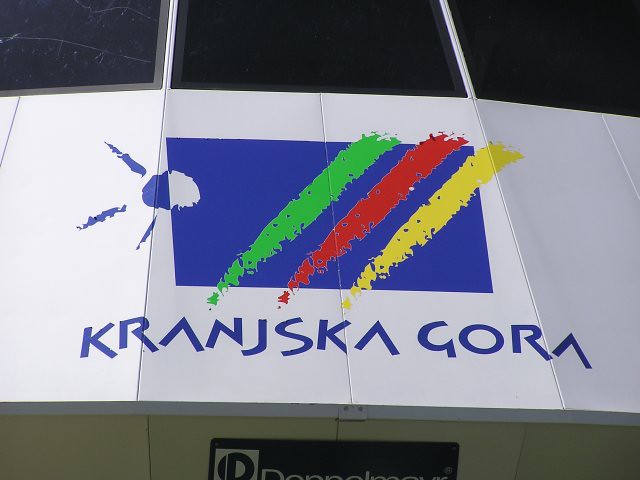In this color photograph, taken in landscape orientation from ground level, we see a close-up view of a white, overhead canopy banner. The central feature of the banner is a striking blue, horizontal rectangle. From the left side of the rectangle, a blue semicircle, representing a sun, extends outward, with three matching blue rays projecting from it. Diagonally crossing the rectangle from the upper right to the lower left are three paintbrush-like strokes, each a different color: green, red, and yellow, in that order. Beneath this vivid logo, the words "Kranjska Gora" are written in capital letters in a modern, somewhat crooked font using blue type. The banner is set against a backdrop of three black windows visible at the top of the photograph. At the bottom, a partially visible black sign displays white letters, adding a contrasting element to the composition. The image overall exudes a realistic, representational style, capturing the essence of the sign with clarity and detail.